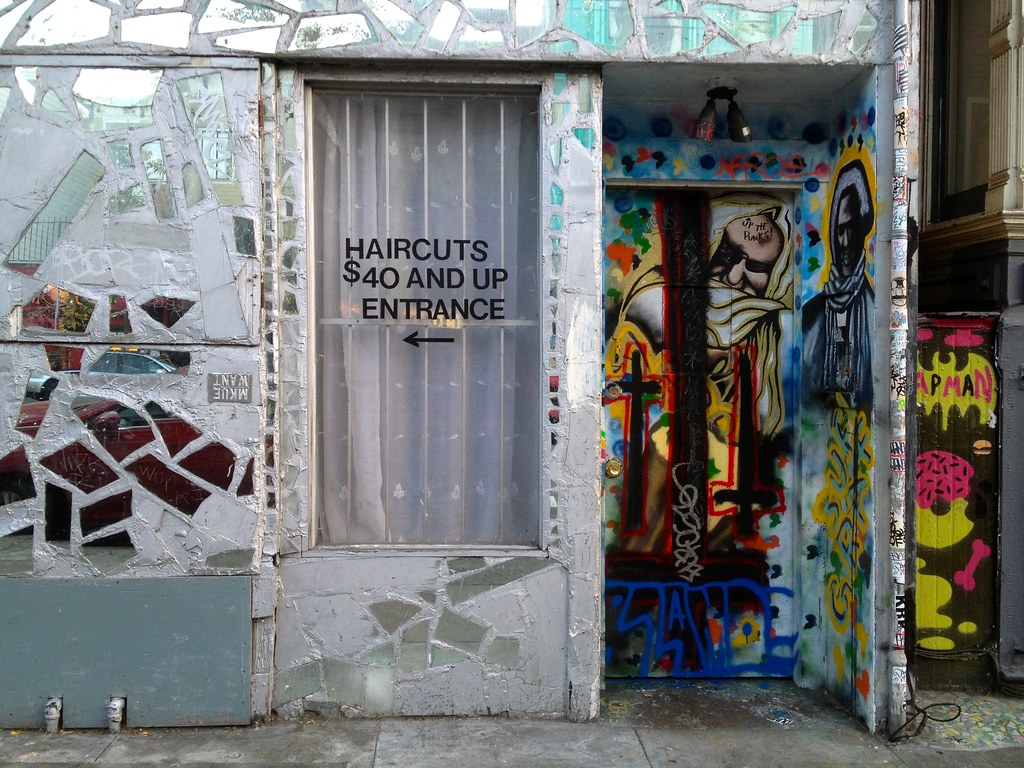The photo depicts the ground level of a city building, possibly located in the Caribbean or a Greek neighborhood. The building itself features an intriguing mosaic façade made of large, irregularly shaped pieces of iridescent glass embedded in concrete, giving off hues of turquoise, light blue, clear silver, and bronze depending on the lighting and angle. This artistic blend of materials is visually captivating.

In the center of the building, there's a clear door adorned with a decal advertising haircuts priced at $40 and up, accompanied by the word "entrance" with an arrow pointing to the left, guiding patrons to the entryway. To the right of this door, there's a doorway that appears to double as a cubbyhole, entirely blanketed in a vibrant mural that has subsequently been overrun by graffiti. This mural likely contains bright colors and historical or religious imagery, including a man with a halo and a cross, partially obscured by tags.

Adjacent to this doorway, along a short wall, more graffiti is visible, featuring playful elements such as a donut, a dog bone, the altered "App Man" Batman logo, and hot pink clouds. This wall borders an alley, further adorned with murals and tags. The sidewalk fronting this scene is concrete, somewhat dirty but not unkempt. This intriguing mix of art and urban decay creates a vivid, dynamic street scene teeming with cultural references and artistic expression.